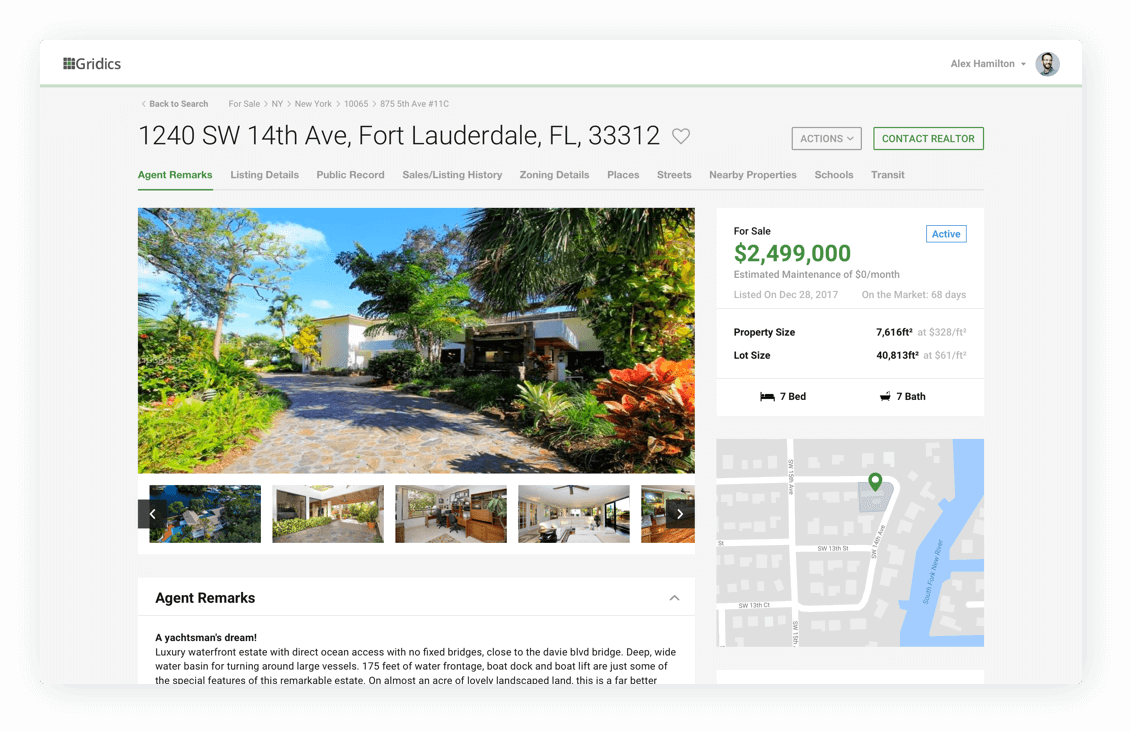**Real Estate Listing Page Overview**

- **Header Section:**
  - The top of the page displays a long white bar.
  - On the far left, there’s a black square comprised of smaller squares, likely a logo.
  - Next to the logo, "Riddick's" is written in black, while on the far right, "Alex Hamilton" is displayed in gray letters. Adjacent to this, there’s a gray dot followed by a circle containing a cartoon image of a Caucasian man with a beard on a gray background.

- **Navigation Path and Property Address:**
  - To the left: Gray text navigation path including "Back to Search," "For Sale," and hierarchical links leading to "NY", "10065", "875 5th Avenue, Number 11C."
  - Below that in large black letters: "1240 SW 14th Ave, Fort Lauderdale, FL, 33312."
  - A gray heart icon and a gray "Actions" dropdown menu sit to the right of the address.
  - An adjacent green-rimmed box reads "Contact Realtor."

- **Interactive Menu:**
  - A clickable menu with tabs in green and gray:
    - "Agent Remarks" (highlighted in green with a gray bar beneath)
    - Other tabs include "Listing Details," "Work Records," "Sales/Listing History," "Zoning Details," "Places," "Streets," "Nearby Properties," "Schools," and "Transit."

- **Property Image and Additional Photos:**
  - A large square image of a tropical property with a clear blue sky, a few clouds, and a stone driveway leading to a white house surrounded by trees, including a visible palm edge on the upper right.
  - Below this main image, there are four smaller pictures showing different views of the house, navigable via arrows.

- **Agent Remarks and Listing Information:**
  - Below the photo, a white bar contains black text: "Agent Remarks."
  - Under Agent Remarks: "Yachtman's Dream" and a partially visible paragraph that’s cut off.

- **Listing Summary:**
  - On the far right: A large white square labeled "For Sale" in green.
  - A blue-rimmed box with white interior and blue text says "Active."
  - The price in green: "$2,499,000"
  - In gray: "Estimated Maintenance of $0/month"
  - Listed on Dec. 28, 2017, and it has been 68 days since listing.
  - Below that, a gray bar displays:
    - "Property size" in black and gray (exact measurements unclear due to small text)
    - "Lot size" details in black and gray text
    - Bed icon indicating "7 bed"
    - Bath icon indicating "7 bath"
  
- **Community Map:**
  - A final square picture shows a basic outline of the community map, featuring white lines for streets, a blue icon for a river, and a green location icon pinpointing the property.